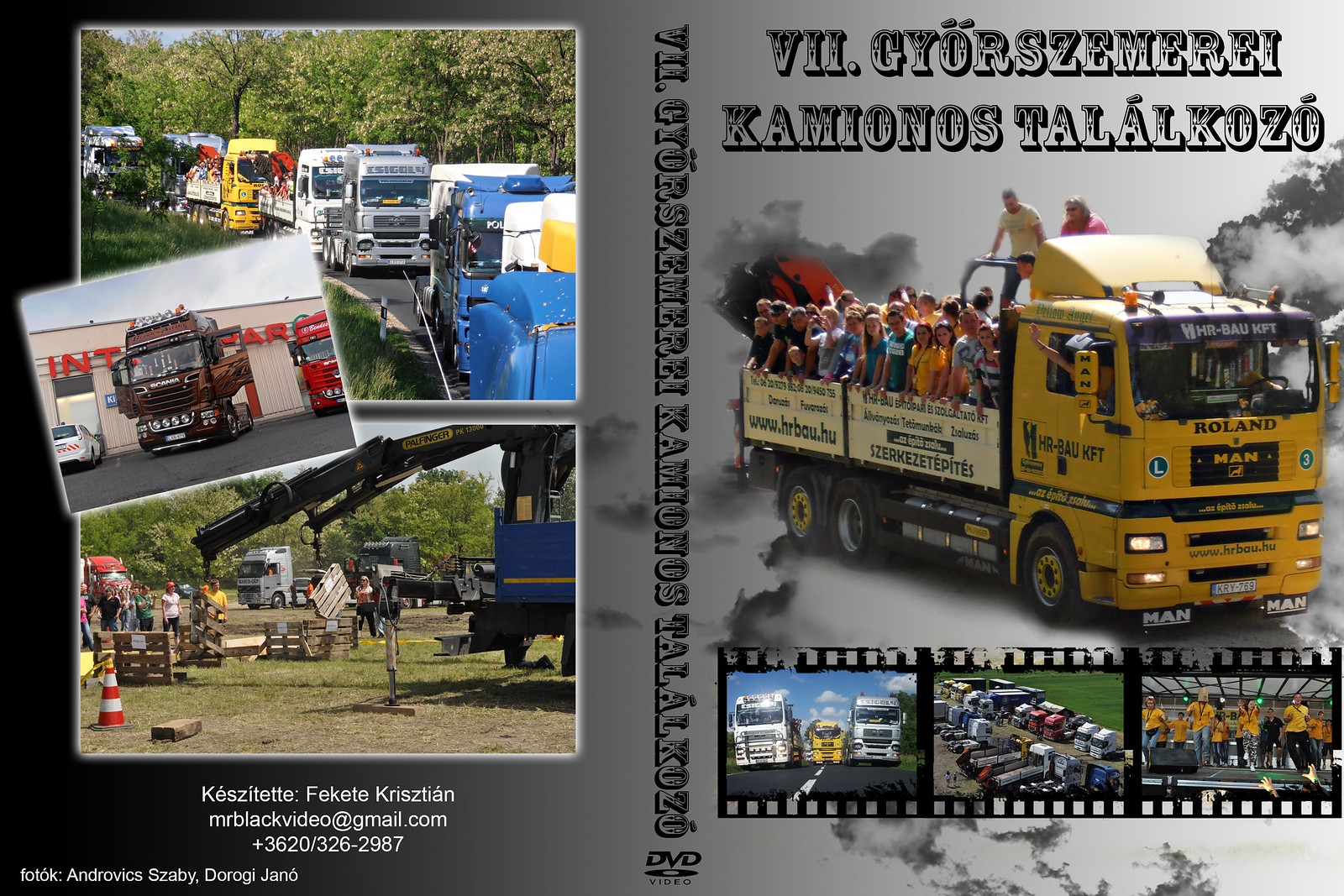The image appears to be an advertisement, possibly for a DVD or an event, featuring various aspects of trucks and truck-related activities. The left side of the image showcases three pictures: two similar-sized images featuring large trucks on tree-lined roads and a smaller angled image depicting either equipment in use with bystanders surrounded by fences and cones or several trucks parked outside a building. The right side prominently displays a large yellow truck labeled "Roland Mann" with people standing in its bed. Below this truck are three smaller filmstrip-like images showing additional vehicles and people, including scenes of trucks on roads, in fields, and possibly workers in a truck factory. The advertisement includes text in a foreign language, with an email address, a contact name, and a phone number provided for further information. The overall theme centers around showcasing different types of trucks in various settings, from parades to construction sites.